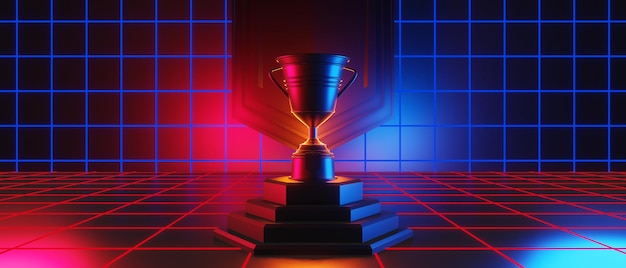The image is a multi-color digital piece featuring a room with no distinctive border or background. The back wall and floor are adorned with a grid of horizontal and vertical lines. The wall transitions between colors, with the far left and right corners in black, moving to blue toward the right center and red toward the left center. The floor follows this pattern, with the right side illuminated in blue and the left side in red, transitioning into blue grout and red tiles on the respective sides. Centrally placed in the room is a four-tiered hexagonal pedestal holding a cup-style trophy with a shield-like object behind it. The trophy, positioned in the middle, catches light that makes it appear red on the left and blue on the right. The lower left corner of the image is bathed in bright pink light, while the lower right corner shines in bright blue light, creating a dynamic and vibrant composition. Also notable is a source of yellow light shining from behind the trophy, adding depth and focus to the scene.